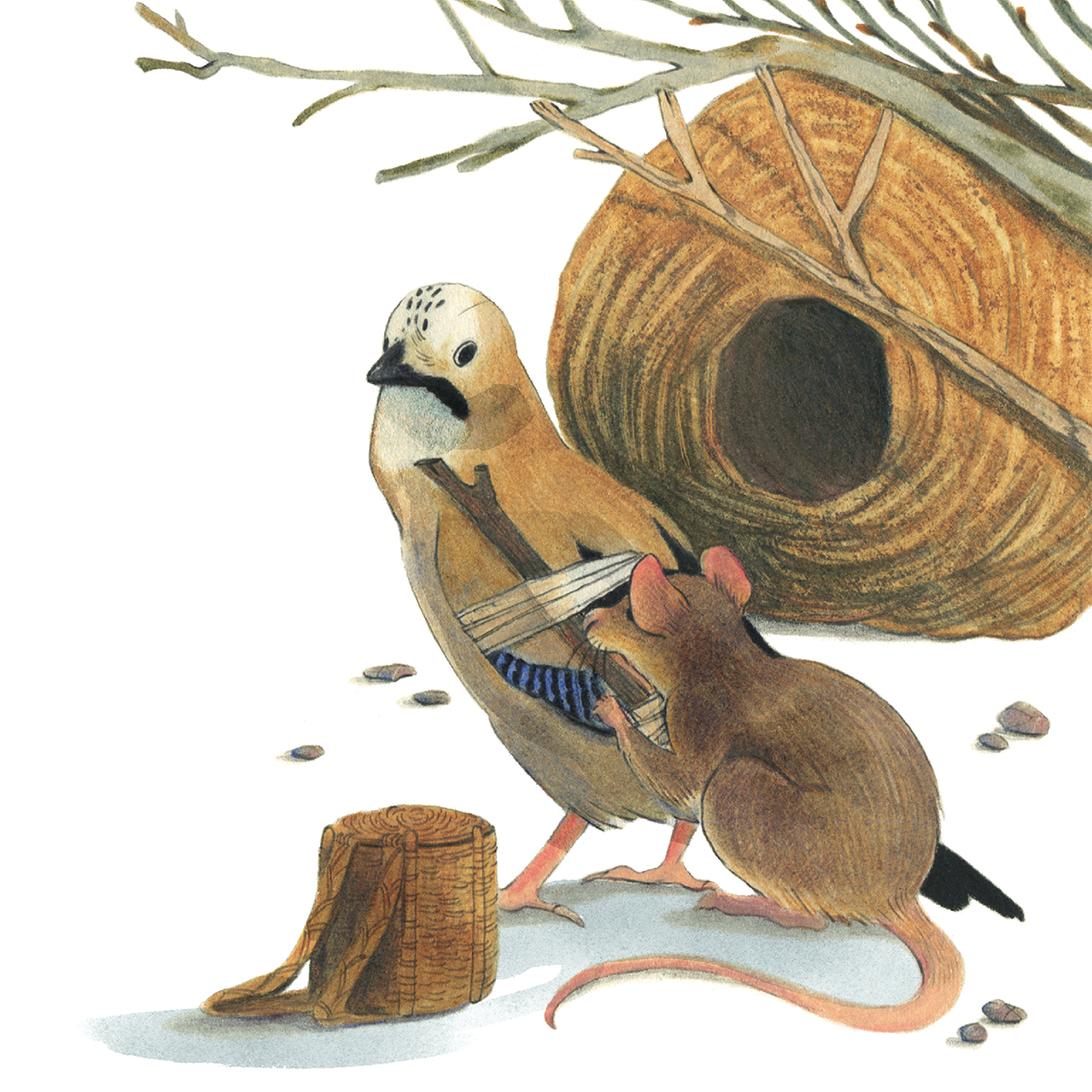The artwork depicts a poignant scene involving a bird and a mouse. At the center of the drawing, a bird with a white face, accentuated by black eyes, and a black beak, exhibits a mix of light brown and cream feathers on its body. The bird appears distressed with a fallen nest nearby, depicted as a circular, beehive-shaped burrow nestled among tree limbs colored in shades of brown and gray.

A compassionate brown mouse, identifiable by its pinkish ears and tail, is positioned to the bird's bottom right. The mouse is tenderly bandaging the bird’s injured wing using a small stick, showcasing a touching moment of interspecies empathy. To the right of this heartfelt interaction, a small wicker basket, likely holding medical supplies, sits beside them. Scattered around the scene are a few pebbles, adding a subtle texture to the otherwise plain white background.